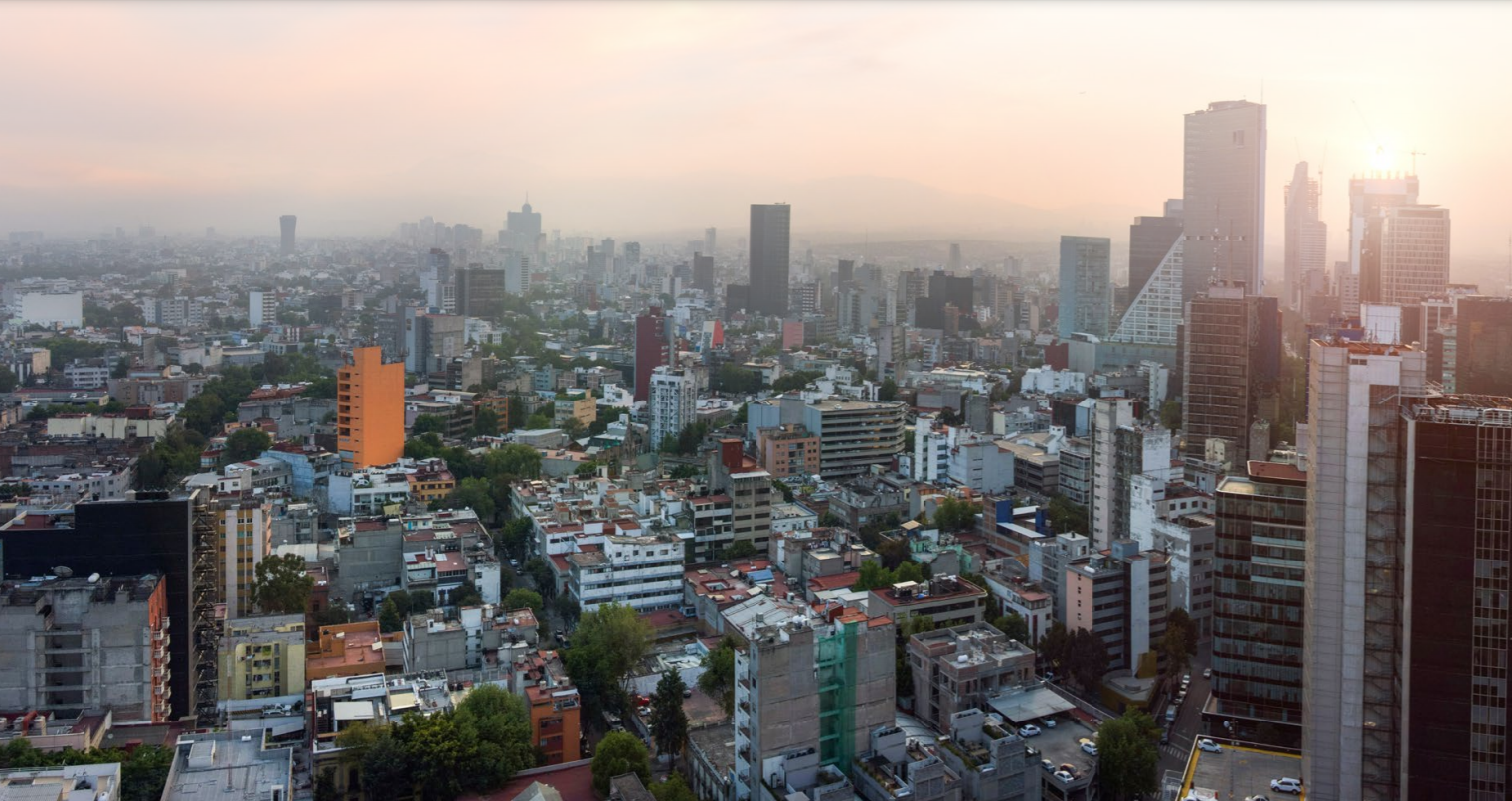A high-altitude photograph captures a sprawling view of Mexico City from the top of a skyscraper. The skyline is dominated by a mixture of very tall office buildings, older and run-down structures, and neglected rooftops cluttered with various items, suggesting they are used as living spaces. The city is enveloped in a thick haze of smog, rendering the distant buildings into mere silhouettes and subtly outlining mountains on the horizon. The sky, painted with hues of light orange, hints at either sunrise or sunset. The streets below are lined with trees and cars, adding a touch of greenery to the urban scene, despite the pervasive pollution obscuring the background.